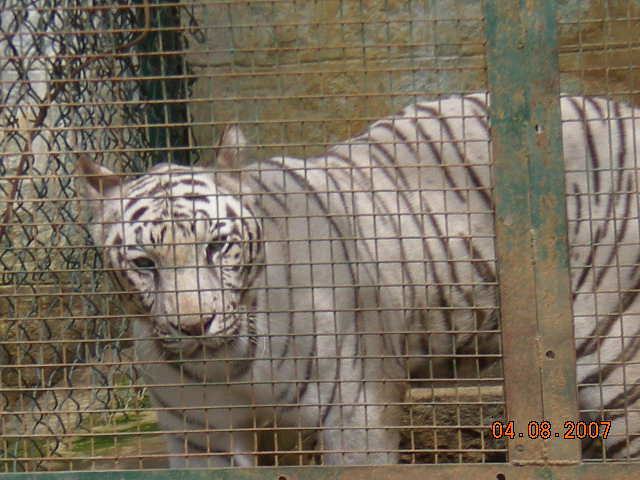The image depicts a white Bengal tiger in captivity, viewed through a sturdy cage made of green and rusted gray metal bars with wire mesh. The tiger, with its striking white fur and narrow black stripes, is positioned with its body in a side profile while its head faces the camera, giving it a direct and slightly disinterested gaze towards the viewer. The setting suggests a zoo or a similar facility, with the background revealing additional chain link fencing and a discolored concrete wall that appears grayish-green, likely from weathering over time. The bottom right corner of the image shows a date stamp reading 04-08-2007 in red text. Despite being confined, the tiger's majestic presence is palpable through the lens.